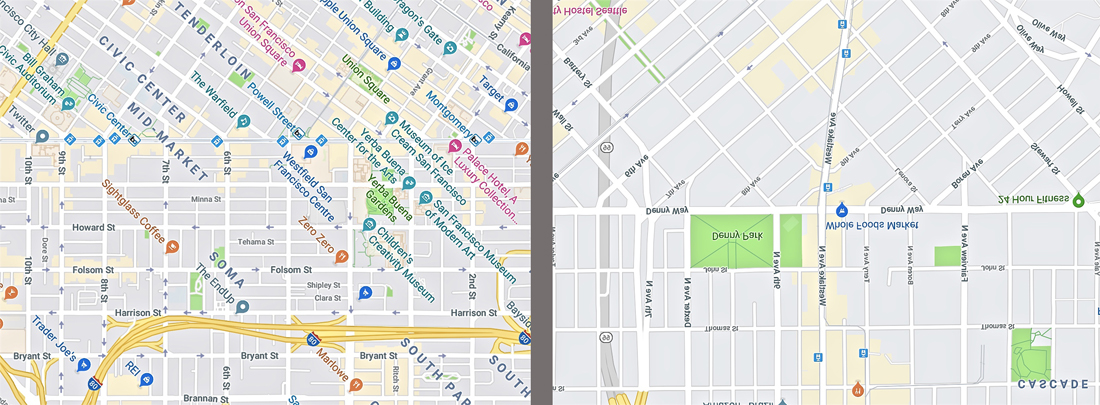The two side-by-side images depict maps resembling navigation or location services. The first map is highly detailed, showcasing a network of roads and numerous pinpointed locations within San Francisco. Notable landmarks and destinations include the Civic Center, mid-Market, Tenderloin, Union Square, Target, Drakens Gate Palace Hotel Luxury Collection, Museum of Ice Cream, San Francisco Museum of Modern Art, Interstate 80, Sightglass Coffee, Trader Joe's, San Francisco City Hall, and Bill Graham Civic Auditorium. In contrast, the second map appears upside down, displaying far fewer locations and labeled in a different language. It provides minimal information compared to the first, highlighting the stark difference between the two maps.